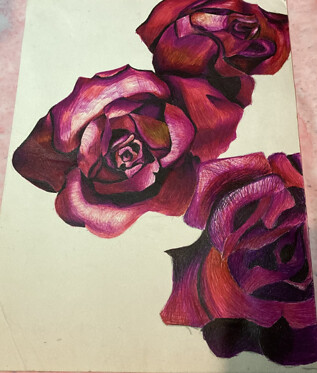A delicate painting on a white sheet of paper lies gracefully against a backdrop of a pink marble or granite surface. The artwork depicts three prominent red roses that appear to be meticulously rendered with colored pencils. The roses are predominantly pink, with subtle hints of orange adding warmth, and touches of black strategically placed to create depth and separation between the petals. The central rose is fully detailed, capturing its entirety, while the upper blossom is viewed from the side, providing a different perspective. The bottom rose, in contrast, is drawn with fewer details, giving a simplified yet elegant representation. The interplay of light and shadow in the coloration brings the roses to life, creating an enchanting visual effect.